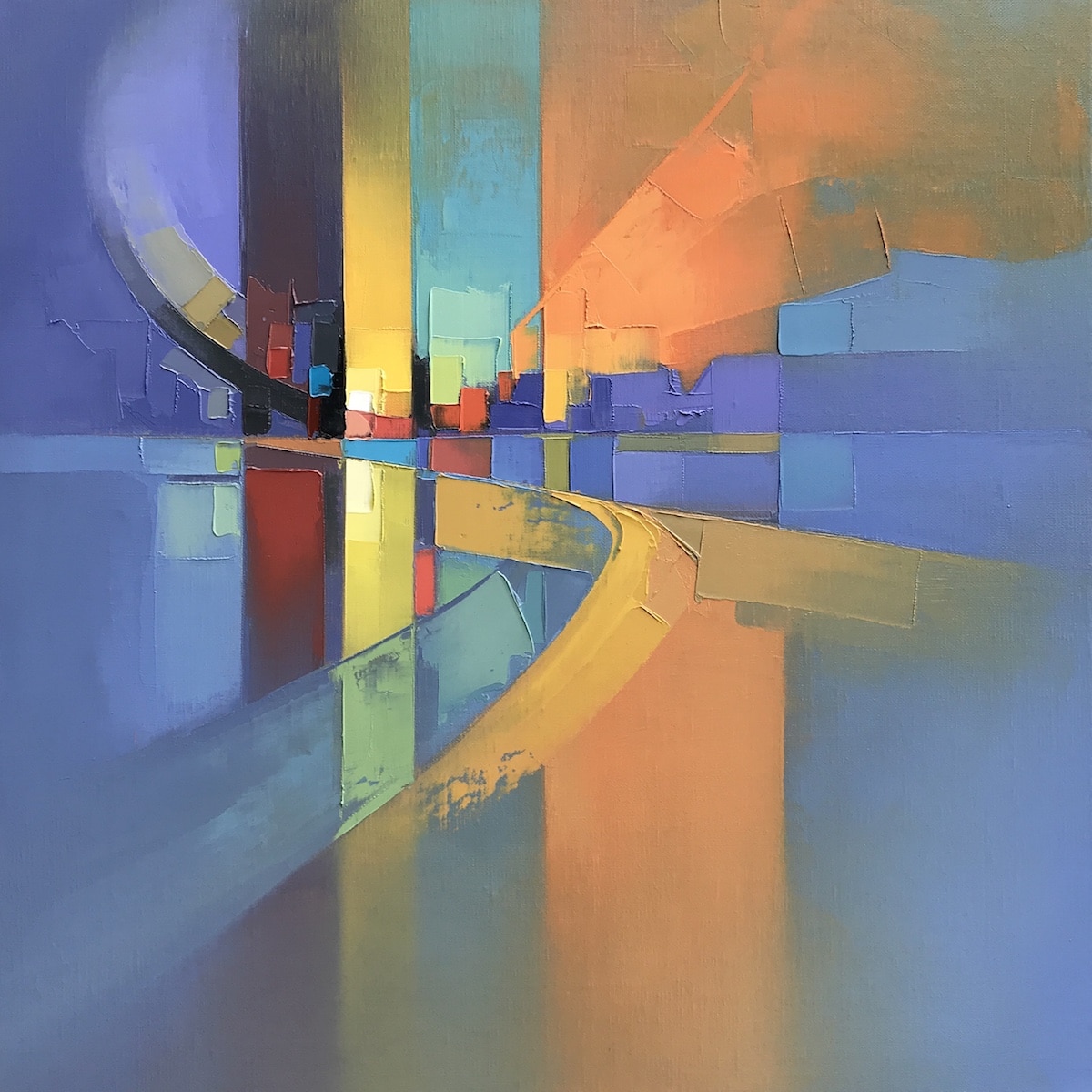The image depicts a detailed abstract painting characterized by thick, chunky layers of paint, potentially acrylic or oil. The dominant color scheme features various shades of blue that encompass the lower right-hand side, upper left, and lower left of the canvas, ranging from cerulean to dark indigo. Towards the middle right of the painting, these blues merge into vibrant orange and yellow hues, forming a central stripe that fades towards the edges. This composition is interspersed with a multitude of vertical and horizontal rectangular and square shapes, creating a suggestion of an abstract cityscape against a horizon line.

Thick layers of paint give the structures a textured, almost three-dimensional appearance, with visible ridges on the edges. The rectangular and square forms display a spectrum of colors including yellow, orange, purple, teal-green, and black, creating a dynamic visual rhythm that suggests reflections in a body of water below. Vertical streaks of color — yellow, purple, orange, and light blue — emanate from the middle of the painting and fade as they reach the bottom, enhancing the illusion of reflective light fading in water.

The upper two-thirds of the canvas are populated with various colored boxes — black, red, blue — further enhancing the abstract cityscape feel. Swirls of yellow and blue paint add a sense of movement and depth, creating a somewhat transparent and swirling effect that merges colors like teal and green, emphasizing the painting's modern and abstract nature. The swirling strokes and the arrangement of shapes evoke an impression of a city at dusk, with its lights reflecting softly on an imagined water surface below, suggesting a serene yet vibrant urban landscape.